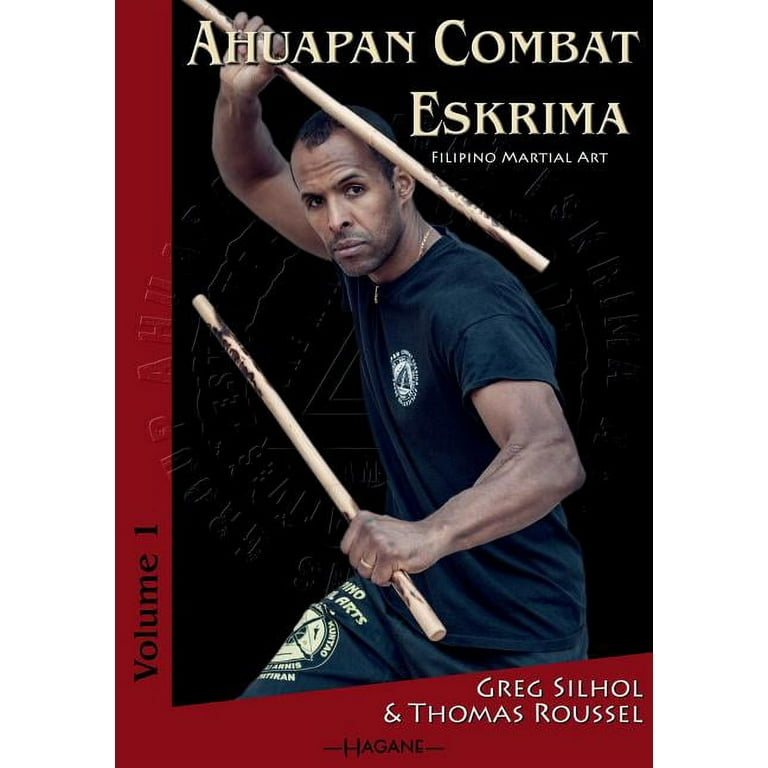The image depicts the cover of a book titled "Ahuapan Combat Escrima," subtitled "Filipino Martial Art." The cover features an African-American man positioned predominantly in the center, dressed in a black shirt and black sweatpants emblazoned with "Filipino Martial Arts" and an emblem, likely representing his studio. He holds two large dowels, approximately two and a half feet long, in a combat-ready stance: his left arm bent with the stick pointing upward toward the left center of the image, and his right arm raised with the stick angled downward over his back shoulder. The background of the cover is black, with a red border along the left side and bottom. The title "Ahuapan Combat Escrima" is written in bold, yellowish text on two lines, with the smaller white text "Filipino Martial Art" underneath. Along the left side, the text "Volume 1" is displayed vertically. At the bottom, the authors' names, Greg Silhol and Thomas Russell, are listed, flanked by dashes with "Hegane" or "Hagans" printed between them. The man is oriented with his body facing to the right but looks directly forward, demonstrating the martial art techniques described in the book.